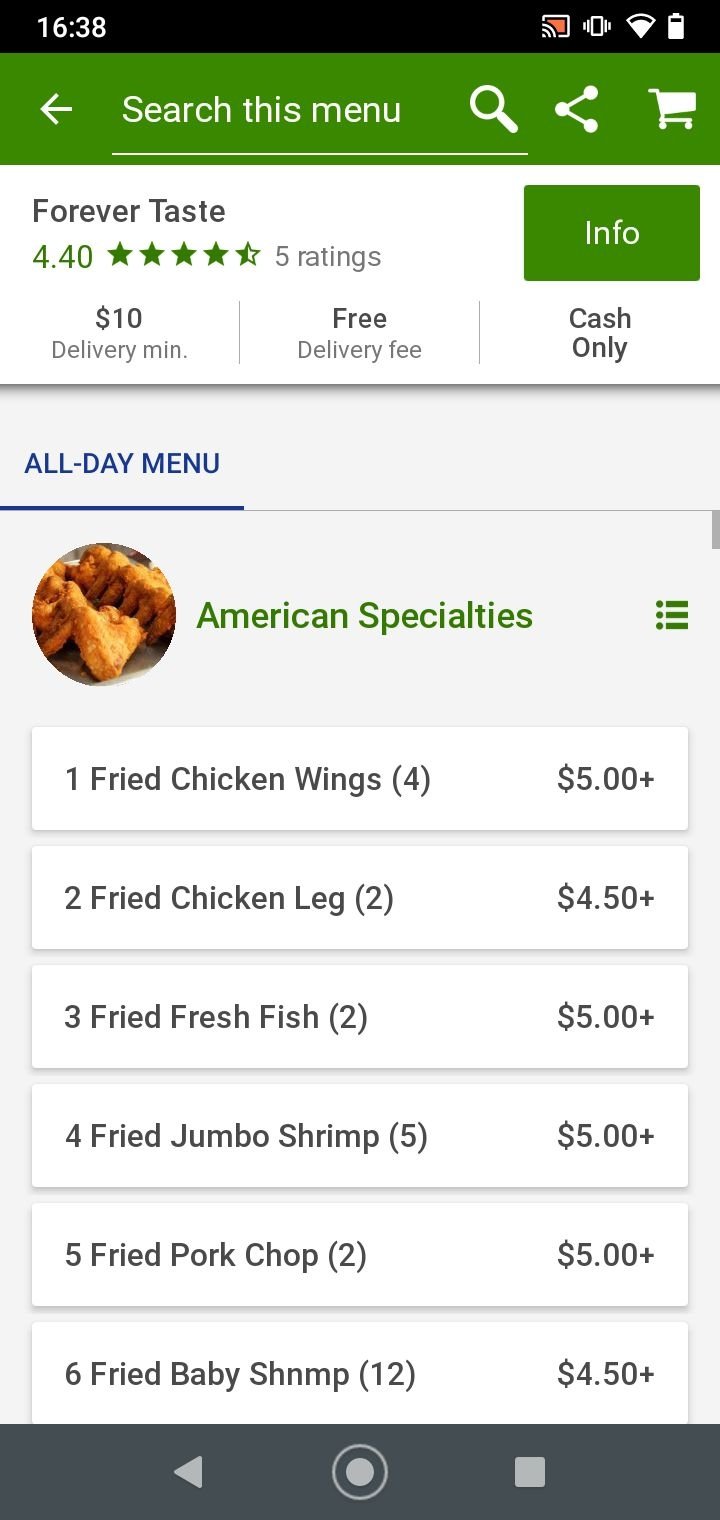In the upper-left corner of the image, the time is displayed as 16:38, while in the upper-right corner, the battery indicator shows it is nearly full in white. Below the time, a long green rectangle with an arrow pointing to the left contains the text "Search this menu" and an adjacent icon of a magnifying glass. Underneath this, in smaller letters, the text "Forever Taste" is presented along with a rating of 4.40 out of 5. An adjacent green rectangle labeled "Info" is prominently displayed.

Further down, the text "$10 delivery minimum, free delivery fee, cash only" is outlined. Below this, in blue underlined text, "All-Day Menu" is visible, accompanied by an image of grilled chicken inside a circle. The green text "American Specialties" follows beneath. Listed menu items include:
- Fried chicken wings (4 pieces) - $5 and up.
- Fried chicken leg (2 pieces) - $4.50 and up.
- Fried fresh fish (2 pieces) - $5 and up.
- Fried jumbo shrimp (5 pieces) - $5 and up.
- Fried pork chop (2 pieces) - Price not specified.
- Fried baby shrimp (12 pieces) - $4.50. 

Each item is detailed with corresponding quantities and prices, providing an extensive overview of the menu offerings.